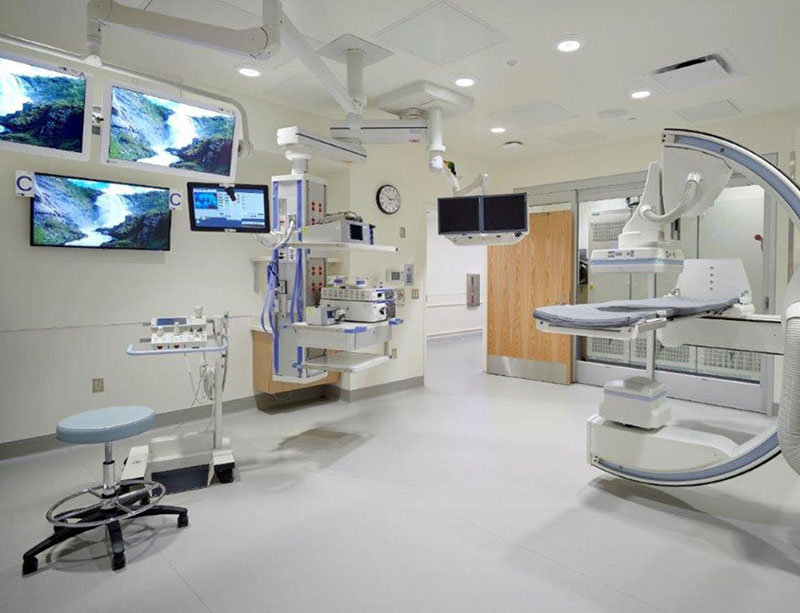The image is a detailed photograph of a high-tech hospital operating room. The center of the image is dominated by a brown wooden door that is propped open, leading to an adjacent area partitioned by a large glass window. The room is filled with advanced medical equipment, including several sophisticated machines clustered in various sections. To the right, there's a narrow patient cot under a C-shaped X-ray machine designed for thorough imaging. The left side of the room features four monitors mounted on the white wall, three displaying identical scenes of an outdoor waterfall, and the fourth showing an unclear image that might depict grass. Below the monitors is a small station equipped for tasks like taking blood pressure, indicated by the presence of a doctor's stool nearby. The floor is a light gray color, and overhead, bright white halogen lights illuminate the room, ensuring visibility for medical procedures. Additionally, a noticeable clock is mounted on the wall, contributing to the room's clinical environment. The abundance and variety of medical equipment underscore the room's purpose for conducting medical tests and scans, confirming it as an advanced operating or examination room within a hospital setting.